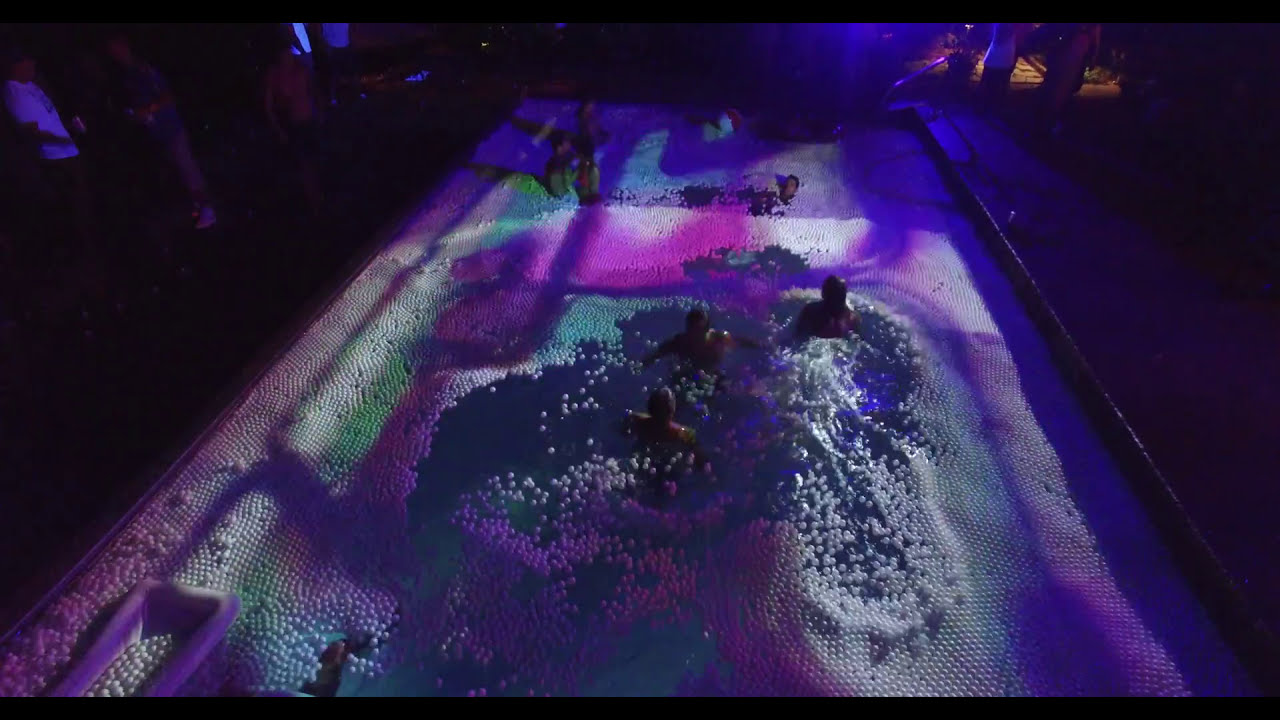The photograph captures an indoor scene resembling a nightclub, illuminated by a striking combination of purple, blue, and green lights. At the center of the image is a narrow, long rectangular pool filled with an abundance of styrofoam balls that mimic bubbles. Approximately eight adults, seemingly in their thirties, are seen swimming amidst these floating balls, suggesting an exuberant, bubble-filled pool party. Around the pool's edge, a few individuals stand holding drinks and engaging in conversation, further implying a social gathering or party atmosphere. The presence of concrete infrastructure, like a surrounding sidewalk, and the distinctive black horizontal bars framing the top and bottom of the image, add to the urban, indoor setting. Overall, the photo exudes a lively and somewhat dark ambiance, characteristic of nightlife festivities.